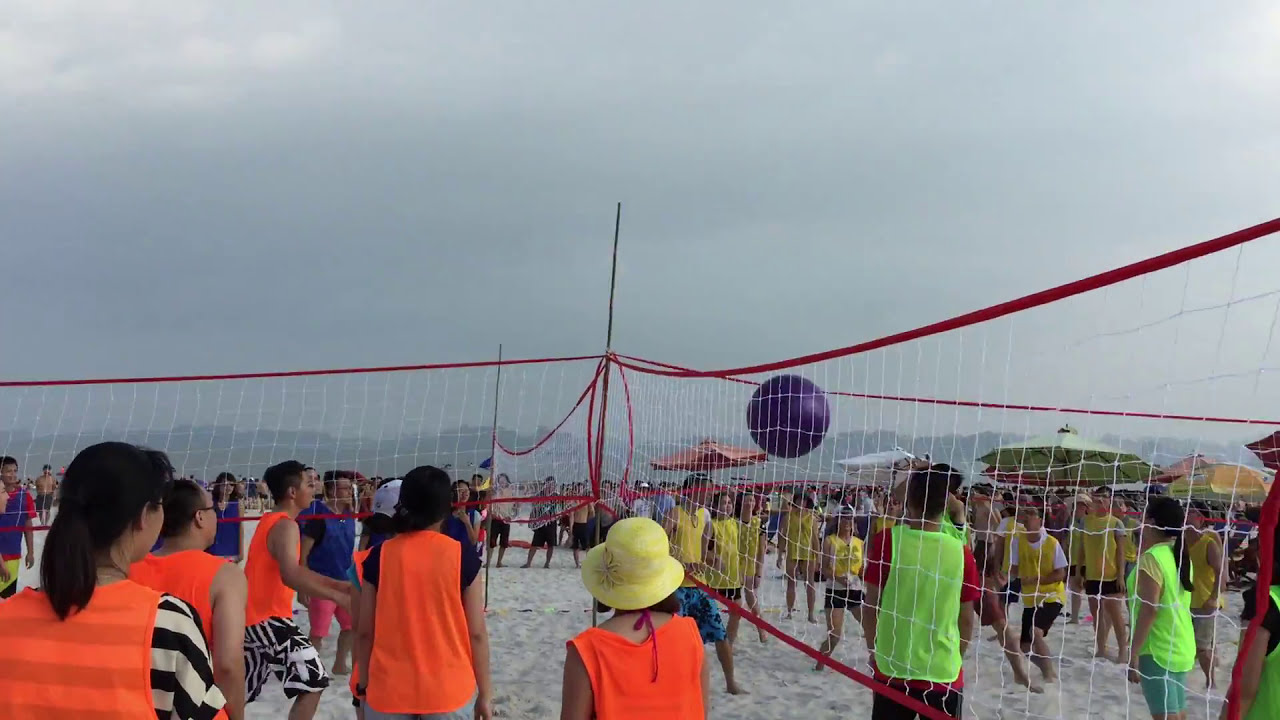The photograph captures a lively scene of beach volleyball with four distinct courts converging at a central pole where four volleyball nets meet, extending in the cardinal directions. The white sandy beach ground is bustling with activity, as teams in different colored pinnies mark the four corners of the frame. In the top left corner, players are clad in dark blue, while the bottom left corner features a team in orange, closest to the viewer. To the right of them, a group is dressed in lime green pinnies, and further to the right, another team is seen wearing yellow. A large blue inflatable ball is prominently suspended in the air, adding dynamism to the scene. Above, a blue sky dotted with white clouds forms the serene backdrop to this energetic setting.